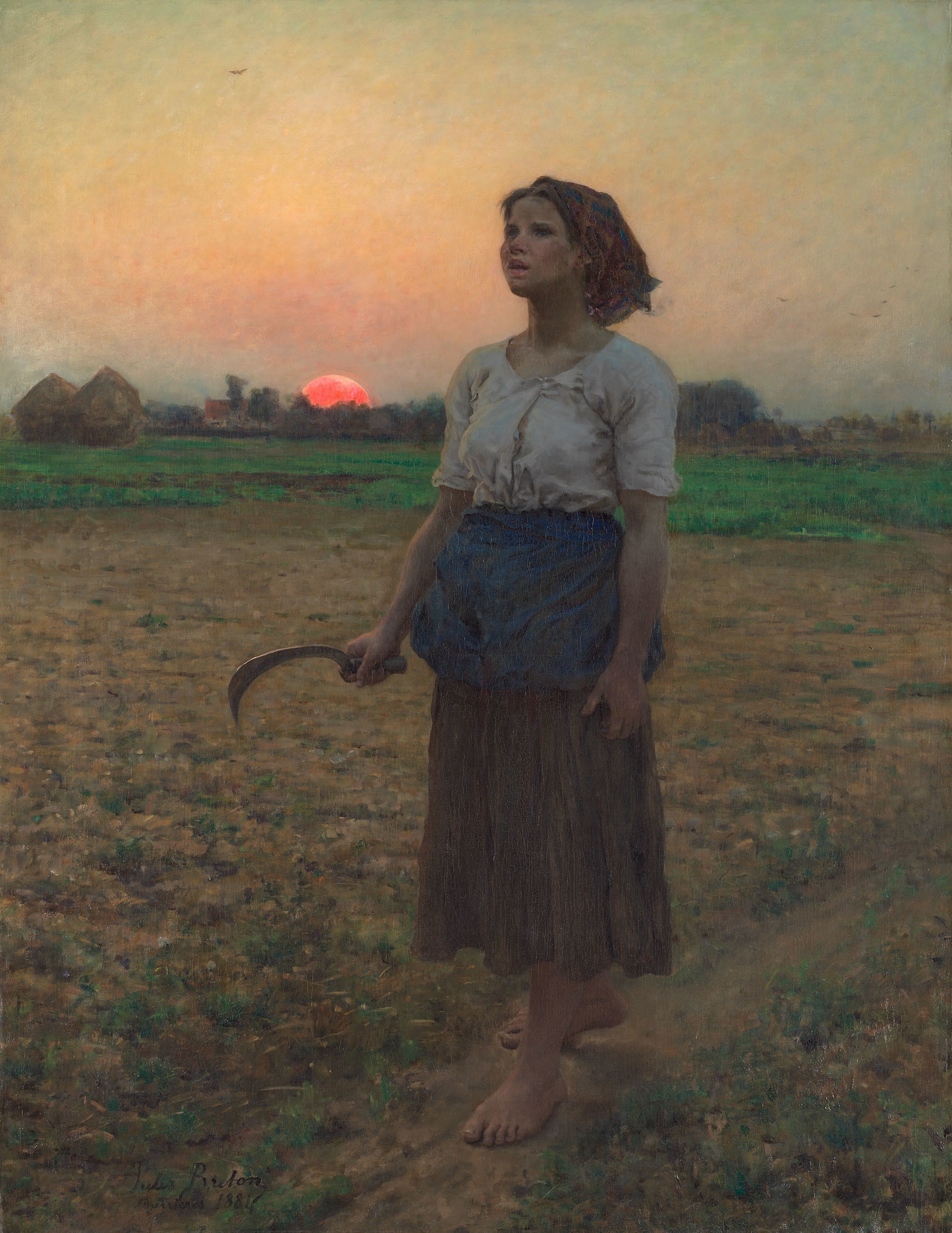The painting depicts a woman standing barefoot on a narrow path through a field filled with green and dead grass. She is in the center of the image, staring off to the left. She wears a brown headscarf, a white short-sleeved blouse, a blue apron over a brown skirt, and holds a gleaming glass sickle in her right hand. Her dark, curved braid ends sharply, adding an element of intensity. The background reveals a serene farm setting with scattered huts and a tangerine orange sun either setting or rising against an orange and yellow sky. The overall scene exudes the warm, earthy tones typical of an oil painting, with a mix of gray from the metal sickle, and various shades of green, brown, and tan accentuating the rustic field. The painting combines elements of solitude and labor, framed in a timeless agricultural landscape.